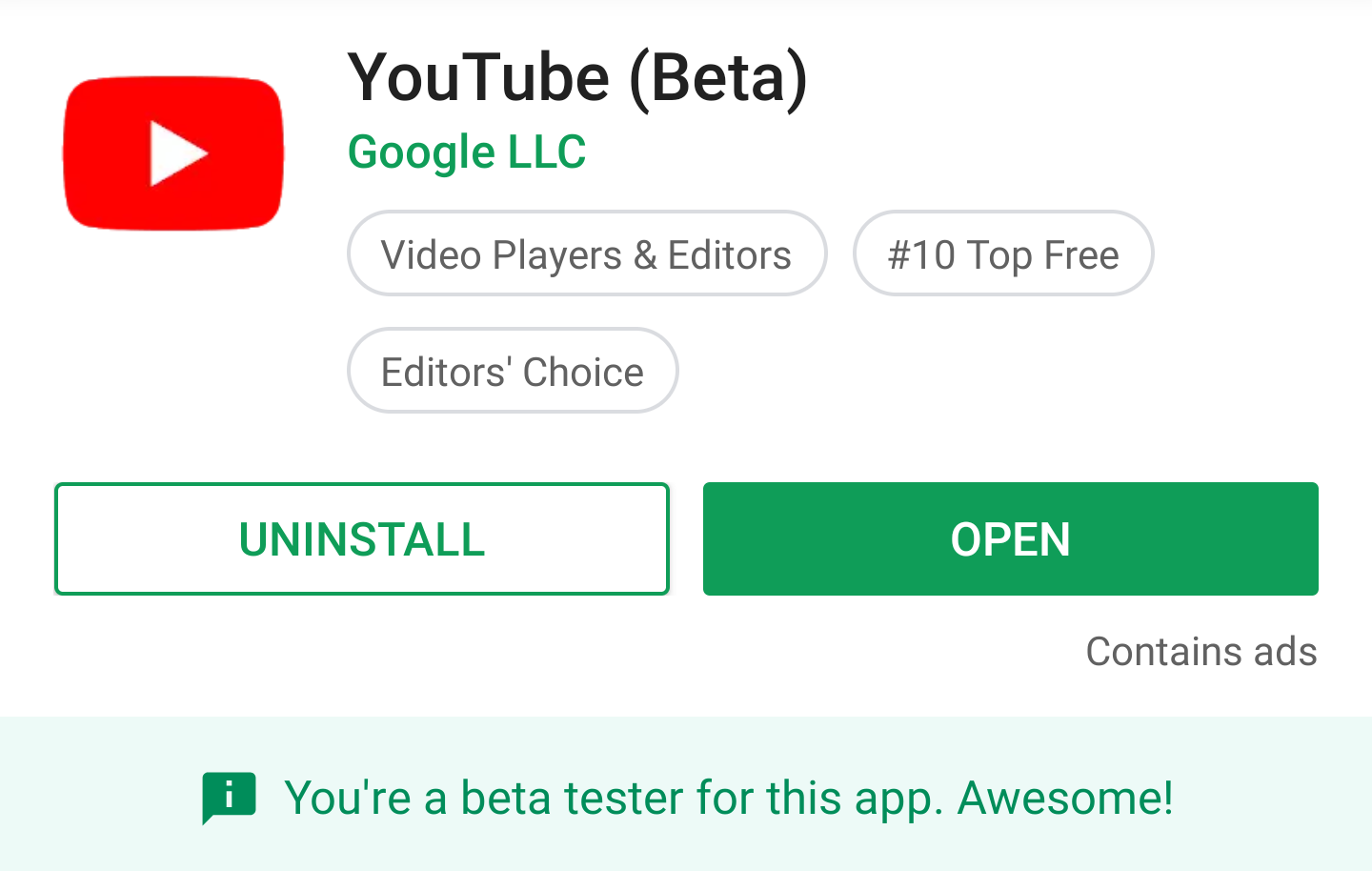This screenshot from YouTube displays the detailed interface of the app's Beta version. At the top, the iconic red YouTube logo with its central white play arrow is prominently visible. To its right, the text reads "YouTube (Beta)." Directly below this, "Google LLC" is displayed in green letters. Further down, bubble callouts indicate the app’s categories, labeling it under "Video Players & Editors." Adjacent to these callouts, "Top 10 Free" and "Editor's Choice" are listed. 

Positioned below these taglines are two action buttons. The left button, outlined in green with green text, reads "Uninstall." The right button, a solid green rectangle, contains the text "Open" in white letters. Following this, a brief note mentions that the app "Contains Ads." Underneath this, a light green banner conveys the message, "You're a beta tester for this app. Awesome." This is accompanied by a small green icon featuring a message bubble with an 'i' inside it.